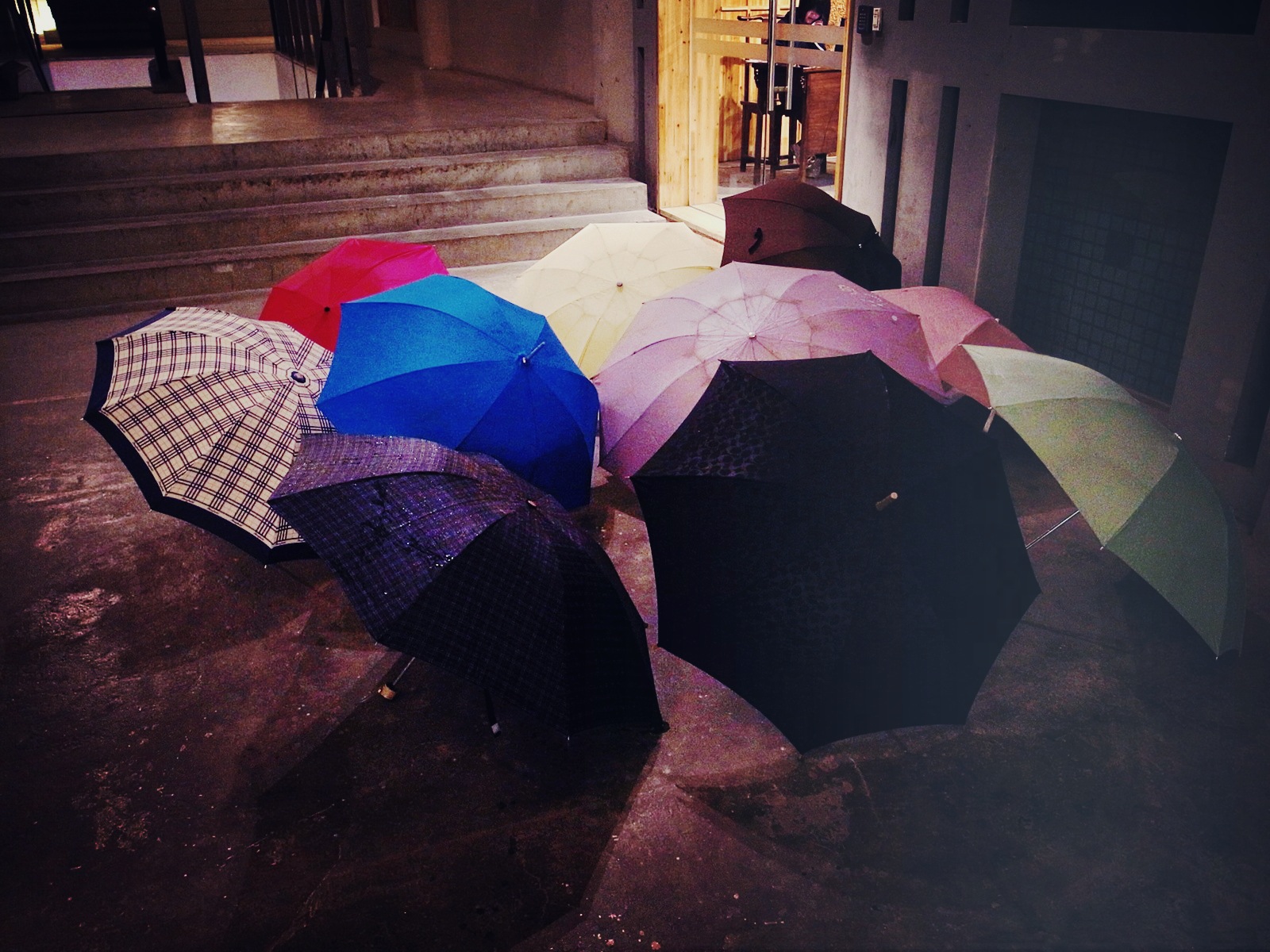In this detailed photograph of an indoor space, possibly an inner courtyard or a public area, we see a collection of umbrellas lying open on a gray, concrete, or stone floor. The background features steps going down and a building to the right with a glass door, which appears to be made of stone. The vibrant array of umbrellas includes various colors and patterns: a yellow one, multiple shades of pink, red, blue, black, white, a beautiful plaid print with a black border, and a distinctive white and black checkerboard pattern. They are all clustered together in the center of the image, resembling a chaotic yet artistic arrangement reminiscent of the tops of balloons. The overall setting and arrangement give the photograph an artistic flair, with the umbrellas forming a visually captivating focal point against the minimalistic backdrop.